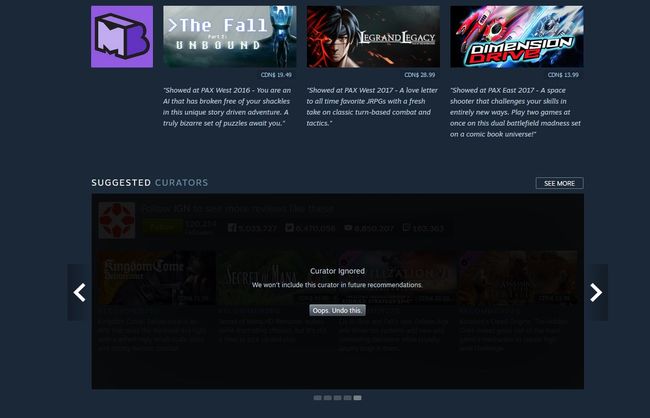Certainly! Here's a detailed, cleaned-up caption for the image described:

"Set against a dark blue background, this image features three game titles displayed horizontally: 'Fall Unbound,' 'Lagrand Legacy,' and 'Dimension Drive.' Below the titles, a purple logo is prominently placed with the text 'Suggested Curators, Curator Ignored' underneath. This indicates that the curator will be excluded from future recommendations. The text throughout the image is primarily rendered in light gray and white, providing a stark contrast to the dark blue background. The games themselves are represented with varying colors, adding visual diversity to the overall composition."